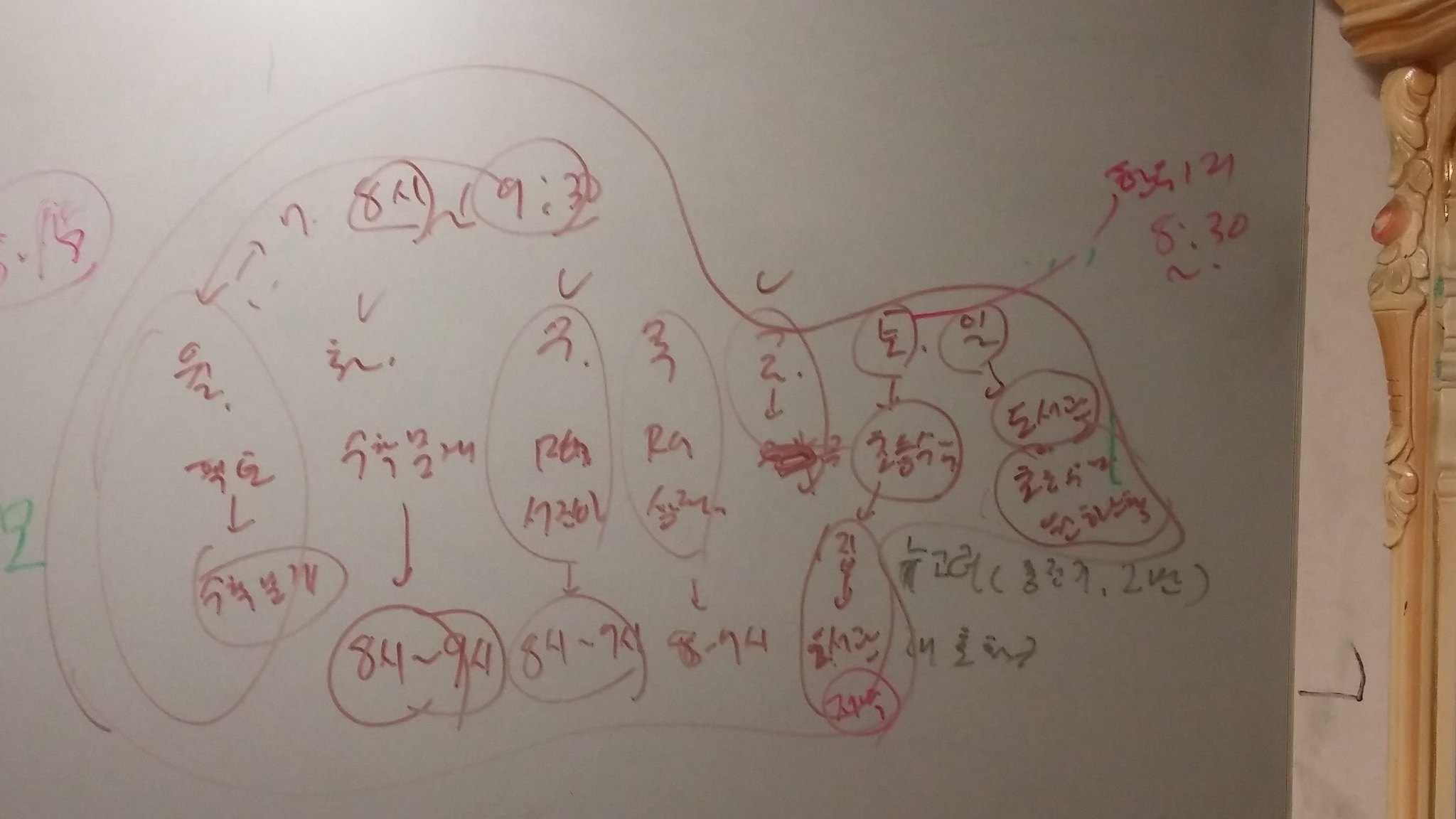Captured in this intricate photograph is a detailed diagram sprawling across a white wall, illuminated by a soft light. The diagram is composed of numerous loops and circles intertwined with a myriad of numbers and symbols, suggesting a complex calculation or mathematical problem. The primary markings are rendered in a bold red marker or pen, with discernible numbers such as 8, 9, and 30, along with various fractions peppering the composition. In the bottom right corner, additional numbers, scribbled in a brown or green marker, offer a stark contrast to the overarching red annotations. The image subtly reveals a corner wall on the right, delineating the edge of the space. Adjacent to this corner, partially obscured, stands an ornately designed light brown armoire, featuring intricate wooden carvings reminiscent of angel wings.